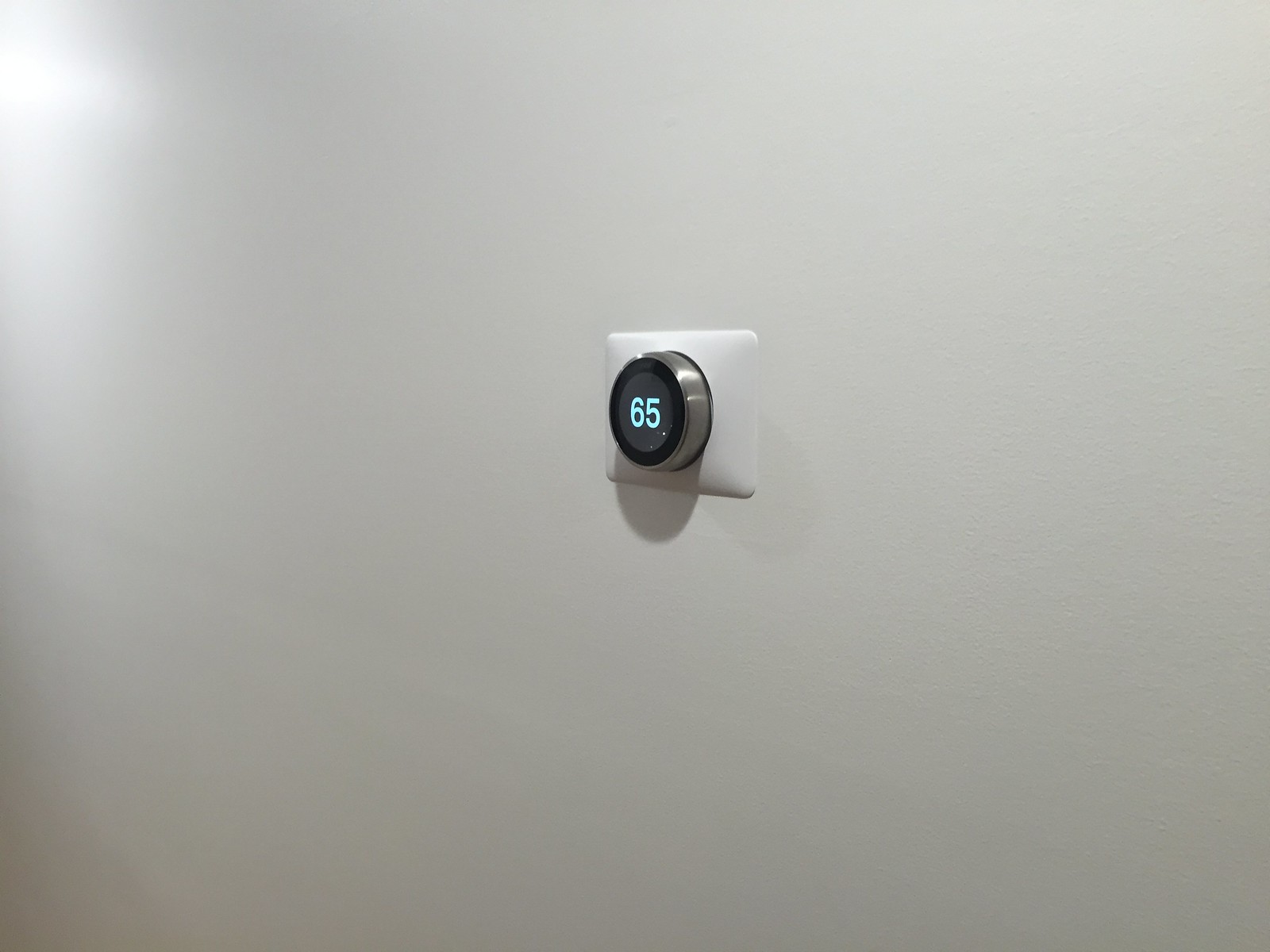This image features a stark, unembellished wall painted in a very light gray or off-white hue, devoid of any spots or imperfections. In the upper left corner, a bright flash of light—possibly from a camera or another light source—creates a noticeable highlight on the wall. At the center-right of the image, there is a square fixture that seamlessly blends with the wall's color. Emerging from this fixture is a round, stainless steel protrusion with a black accent, giving it a modern, sleek appearance. In the middle of this protrusion, a digital dial with a dark gray display shows the faint blue numbers "65." Beneath the round element, a subtle gray shadow falls against the wall, further emphasizing the fixture's presence.